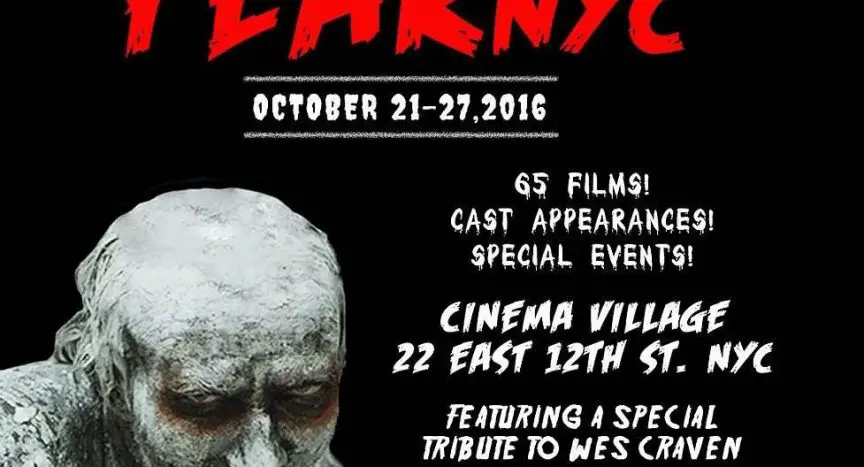The image is a partial piece of a flyer or advertisement for a horror-themed event. The base color is pitch black, with striking details that hint at an eerie atmosphere. In the lower left-hand corner, there's a spooky individual, mostly shown from the nose up. This figure is covered in a thick layer of white paint, with darker, burnt orange or dark gray patches around and leaking from the eyes, giving a rusty, decayed look. Their hair is similarly coated with the white paint, enhancing their ghostly appearance.

At the top of the image, there's vivid red text that seems to say "Fear NYC," but it's cropped off, making it difficult to read the full title. Below, in a white, dripping blood-styled font, the text lists event details: "October 21st to 27th, 2016," followed by "65 films, cast appearances, special events." The text continues with the venue information: "Cinema Village, 22 East 12th Street, NYC." The poster concludes with a special note: "Featuring a special tribute to Wes Craven." The overall design emphasizes a spooky and mysterious theme, perfect for a horror film event.